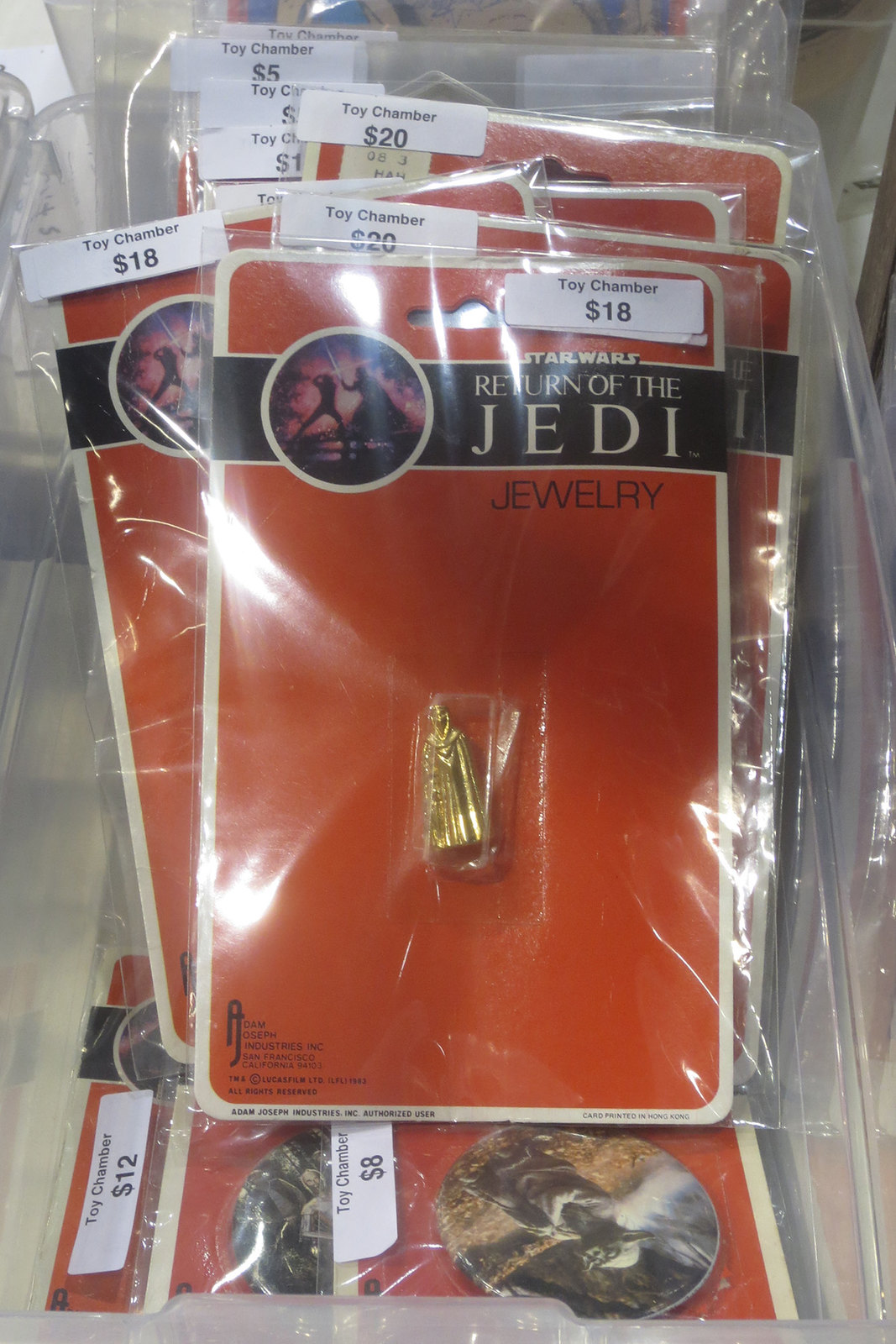The image displays a retail rack containing various Toy Chambers from the Star Wars: Return of the Jedi series. Each Toy Chamber is individually wrapped in a poly bag and includes a red rectangular card with white borders. The card features a black bar with the text "Return of the Jedi" in white letters and a circular image that appears to depict a scene involving Darth Vader. The Toy Chambers, some in gold, showcase miniature figurines and jewelry items related to the movie. Prices are clearly marked on white stickers for each item, ranging from $5 to $20, with noticeable tags showing $18, $20, and $8. All the items are arranged against an orange background, maintaining a consistent font and design theme throughout the display.